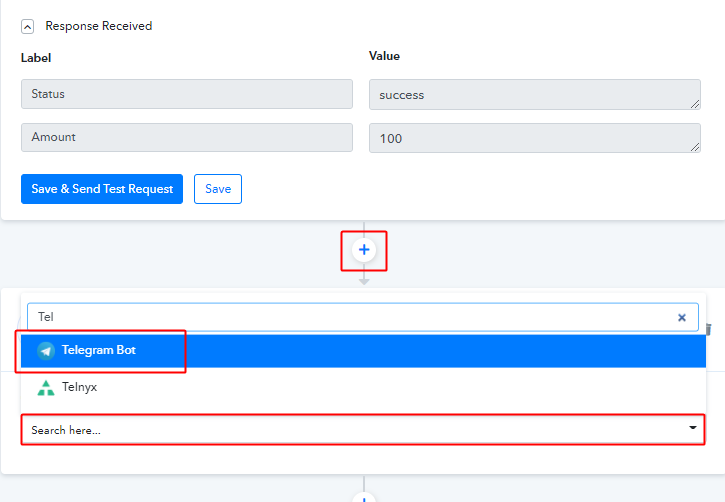In the upper left corner, a small square with a light gray border and rounded edges houses an arrowhead pointing rightwards and upwards. Inside the square, black text reads "Response Received." Below this, bold black text displays "Label."

Beneath the label, there are four editable fields with light gray backgrounds. These fields are labeled as follows:
1. Status
2. Amount
3. Success
4. 100

To the right of these fields, a bold black heading states, "Value for the Success in 100 areas."

Towards the bottom left, a large blue rectangular button bears white text that reads "Save and Send Test Request." Adjacent to this, on the right, a small rectangular icon features a blue outline and blue text that reads "Save."

Further down, a light gray background area features a centered gray arrow pointing downwards. Directly below this arrow, a circular white area with a blue plus sign in the middle is highlighted by a red-bordered square.

Following this, another rectangular white area contains a field currently selected and highlighted with a blue border. This field is labeled "Telegram Bot," and it is framed by a red rectangular border. The blue background of the field indicates its active status.

Finally, underneath this section, a small green triangle with a white "T" in the center is labeled "T-E-L-N-Y-X."